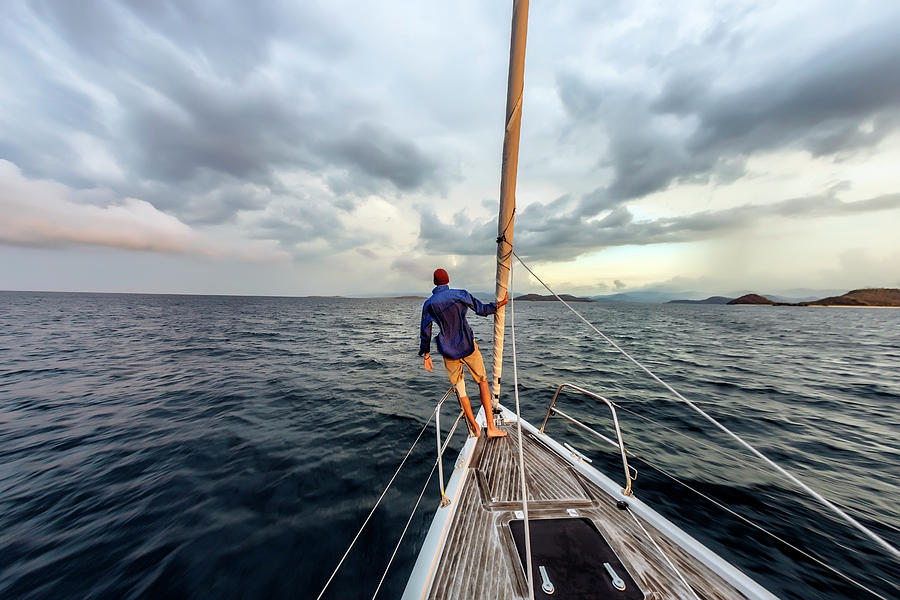In this detailed and photorealistic image, a man is seen on the deck of a sailboat that features a wooden deck and white railings. He is leaning slightly over the port side (left side) of the boat, straddling a thin railing in a position that seems slightly unnatural, suggesting either an unusual angle or possible AI manipulation. The man is holding onto the mast, wearing a red cap, a blue windbreaker jacket, and khaki-colored shorts. His skin has a pale tan, and he is barefoot. Additionally, a wrapping can be seen around his left knee. The background depicts a vast, open body of water, with distant small, hilly islands visible to the far right. The sky above is bright and somewhat cloudy, with a yellow sun partly obscured by the clouds, indicative of mid to late afternoon. The scene converges towards a vanishing point in the center, giving an almost surreal feeling as the sea and clouds appear to draw the viewer's eye inward. The day seems to be slightly stormy, with some waves visible in the otherwise calm sea.